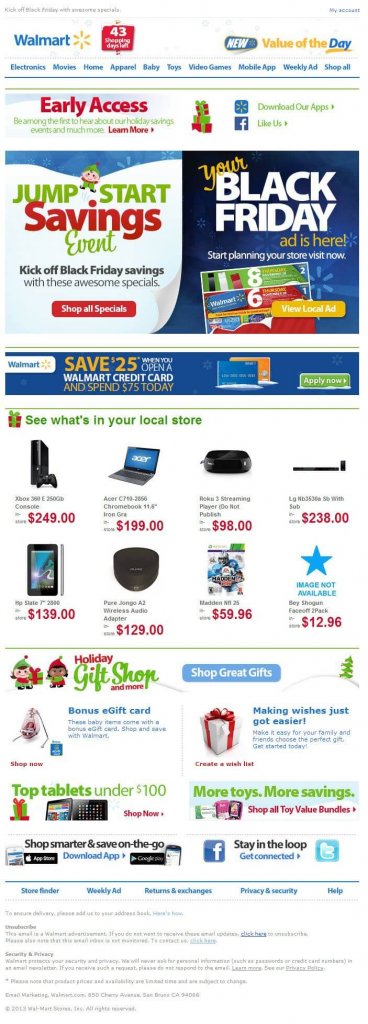The image prominently displays the Walmart logo in blue text accompanied by a gold star at the top. Adjacent to the logo are 43 shopping bags, indicative of a post-holiday, Black Friday-themed advertisement. Below the logo, a navigation menu in blue text offers various category links: Electronics, Movies, Home, Apparel, Baby, Toys, Video Games, Mobile App, Weekly Ad, and Shop All. The top portion also highlights early access for holiday savings announcements, social media links, and an image of stacked Christmas gifts.

The ad transitions to information about a "Jumpstart Event Savings" with a preview for Black Friday deals, encouraging customers to start planning their store visits. There's a promotional offer of $25 off when opening a Walmart credit card, prominently displayed next to images of two laptops, along with a link to apply for the credit card.

At the center of the image, various products are showcased: an Xbox console, a laptop, a Roku player, and a small speaker. Below this section, additional products such as an HP tablet, a wireless adapter, a Madden video game, and a note indicating "Image not available" for a Face-Off 2-Pack Shogun, which appears to be some form of collectible cards.

Further down, the ad promotes the Holiday Gift Shop, highlighting bonus gift cards and featuring imagery of elves and Christmas presents. There is an advertisement for tablets priced under $100 and a mention of more toys and savings. Social media links for Facebook and Twitter and an option to download the Walmart app are provided, encouraging users to shop and save on the go.

The bottom portion includes a secondary navigation menu with options such as Store Finder, Weekly Ads, Returns and Exchanges, Privacy and Security, and Help. The image concludes with fine print containing specific notes and disclaimers.